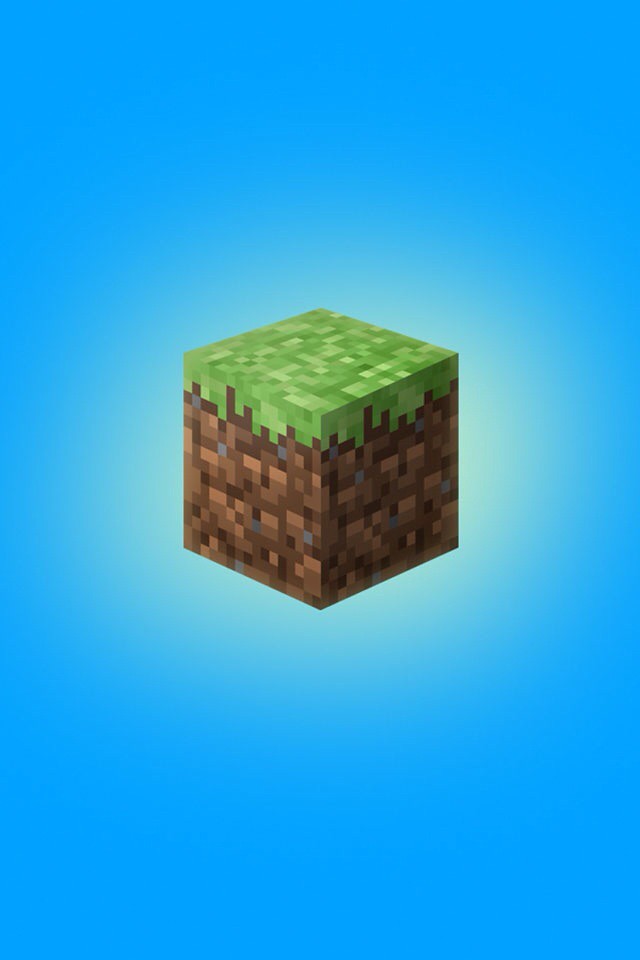This image showcases a three-dimensional, computer-generated model of a cube, viewed from a slightly elevated angle, allowing three of its faces to be visible: the top, and two adjacent sides. The top surface of the cube is rendered in various shades of green, representing grassy terrain, while the remaining 80% of the cube is colored in varying hues of brown, simulating layers of soil and rock beneath the Earth’s surface. Occasional streaks and patches of blue can be seen embedded within these brown layers, possibly indicating underground water or geological features. Overall, the design resembles an educational cutaway illustration of the Earth, akin to those commonly used in physical science classes to demonstrate geological strata.